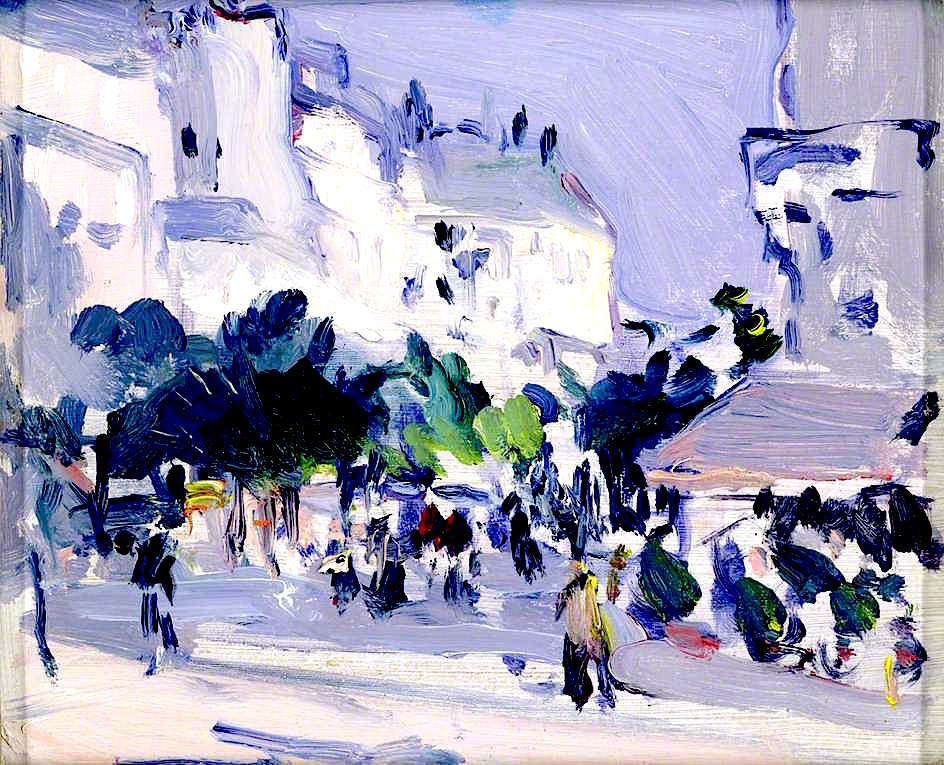This detailed acrylic painting depicts an abstract outdoor winter setting in a small town. Dominated by white, gray, and purple tones, the scene suggests a wintry atmosphere with blurry brush strokes contributing to an overall ethereal quality. In the background, a European-style dome building stands out, its white structure imbued with purple and blue hues. The foreground and middle ground feature indistinct figures walking along a street. These figures, rendered as vertical blobs in various colors, add a layer of human presence to the otherwise serene landscape. Notable colors include yellows, browns, greens, blues, and whites, with one figure displaying distinct yellow-brown hues and contrasting black and blue legs. Green trees and foliage of mixed greens, blues, and oranges add a festive undertone to the scene, lining the sides of the street and creating a sense of depth and vibrancy. The left side of the image is dominated by tall white structures, while the right side features an outline of another building, possibly set on a different-colored curb, adding to the town's charming layout.